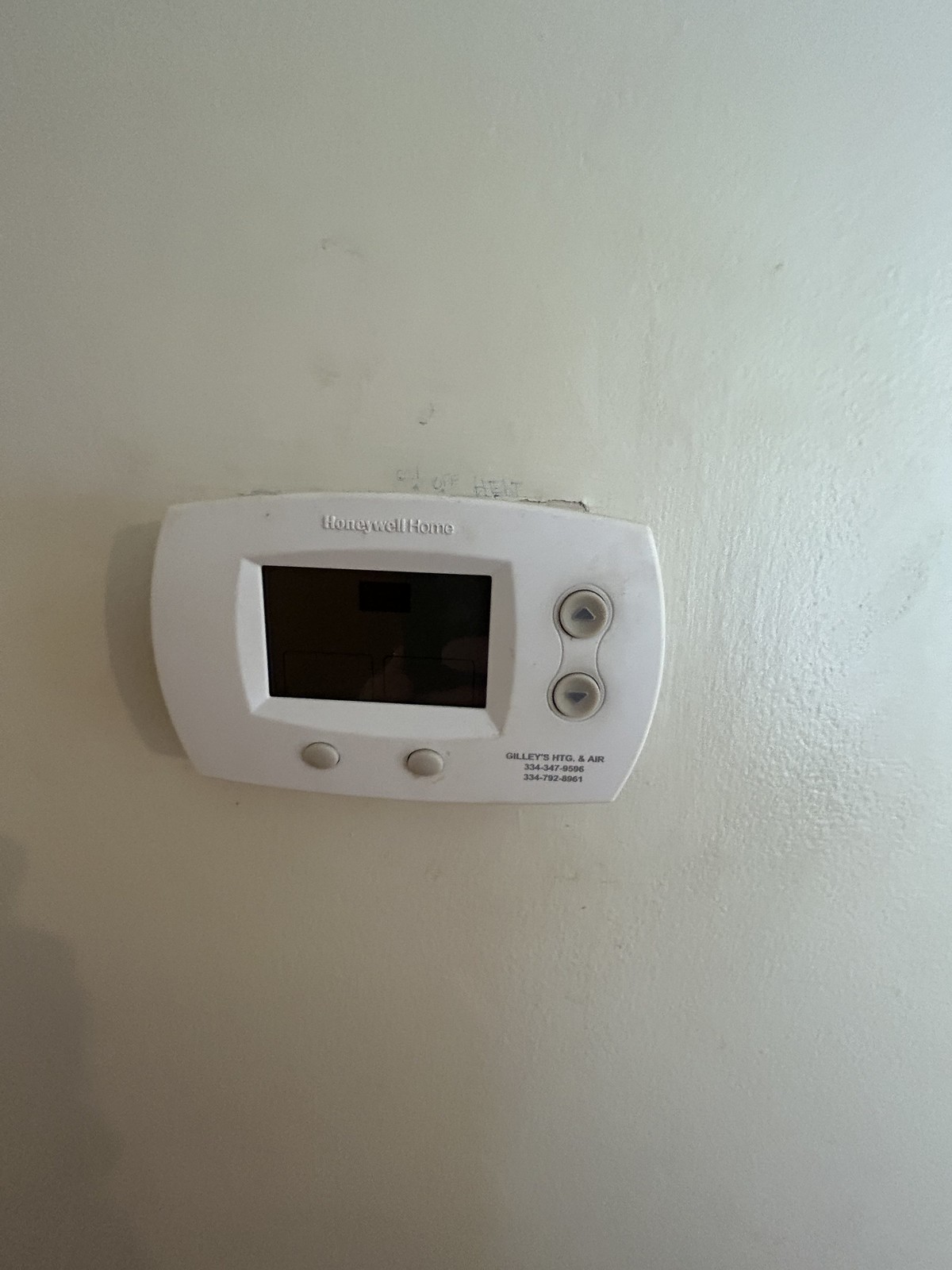The image depicts a carbon monoxide detector affixed to a wall. The device is white with a central black square display. Positioned below the display are two small gray buttons. The top of the device proudly bears the brand name "Honeywell Home." Along the side, there are two circular buttons aligned vertically; the top button features an upward arrow, while the bottom button displays a downward arrow.

At the bottom of the detector, the text "Gillies MTG and Air" is prominently displayed, accompanied by two phone numbers: "334-347-0506" and "334-792-0061." The device appears securely bolted to the wall, which has visible markings and fingerprints, suggesting regular contact or wear. The wall itself shows uneven paint and signs of age, reflecting it is not in pristine condition.